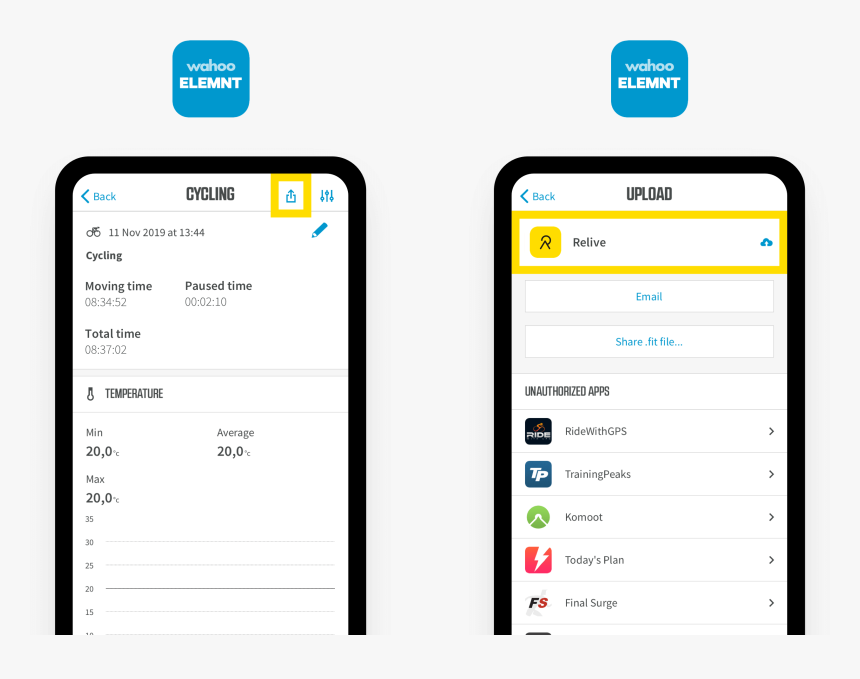Under the "Website" category, there are two images displayed side by side on a light gray background, each resembling a phone screenshot.

The image on the left features a blue square labeled "Wahoo Element." The top of this image includes a navigation option "Back in blue" to return to a previous screen. Immediately below, the word "Cycling" is displayed, followed by a prominently positioned yellow "Upload" button. Underneath, there is a small bicycle icon with the date "11 November 2019" and the time "1344" next to it. An editing pen icon is also visible. Further details include a breakdown of cycling activity: 
- "Moving Time: 834.52"
- "Pause Time: 210"
- "Total Time: 837.02"

A blank temperature section is indicated by an icon of a thermometer, with additional metrics showing:
- "Minimum: 20"
- "Average: 20"
- "Max: 20"

The second image highlights an "Upload" function and includes a similar back navigation button. It is titled "Relive" and features various sharing options such as:
- Email
- Share Fit File
- Unauthorized Apps

The image also lists compatible platforms for sharing:
- Ride with GPS
- Training Peaks
- Today's Plan
- Final Surge